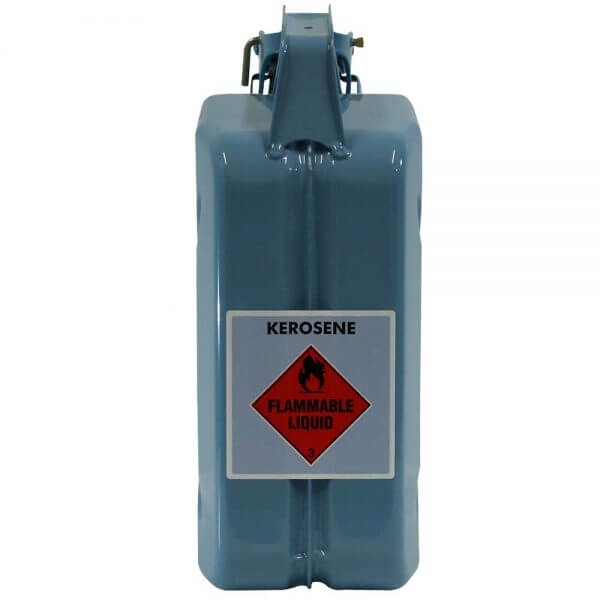The image depicts a shiny, gray rectangular kerosene container standing vertically against a plain white background. The container features a handle and a nozzle at the top and includes a vertical groove running down its middle. Centered on the container is a prominent label: at the top of the label, "kerosene" is printed in bold black, capital letters. Below this, the label consists of a red diamond shape with a black-outlined flame icon. Underneath the flame, the label reads "flammable liquid" in black text. The diamond also includes the number "3" at its bottom. The detailed image of the container captures its metallic sheen and the specific design elements of its warning label, making it clear that this is a kerosene tank meant for careful handling.